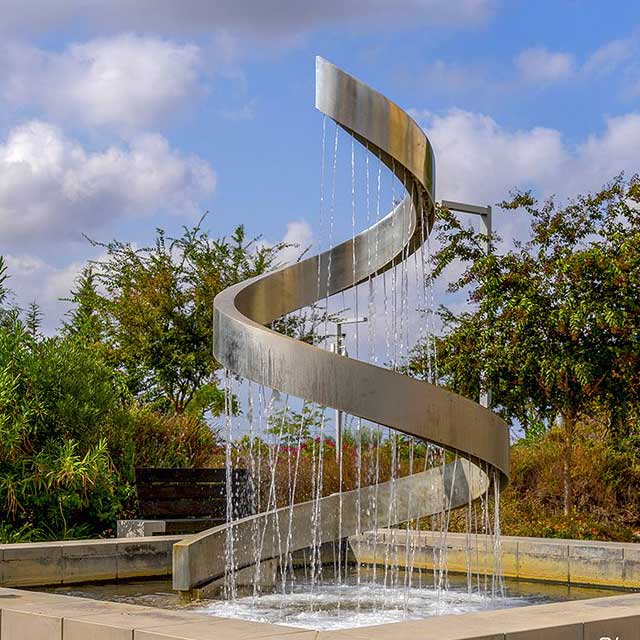This photo showcases an impressive modern outdoor sculpture that doubles as a fountain. The sculpture, crafted from stainless steel, features a striking twist of metal resembling a swirly ribbon or section of a spring. Water elegantly streams out from various points along its edges, cascading into a square pool below, which is bordered by tan stones. In the background, a dark brown bench invites visitors to sit and admire the piece, set amidst green trees and dry orange shrubs. The scene is set under a partially cloudy sky, with areas of bright blue peeking through. The area is illuminated by two modern street lights, adding to the contemporary aesthetic of the sculpture. This beautifully detailed fountain stands out as a centerpiece in its serene surroundings.